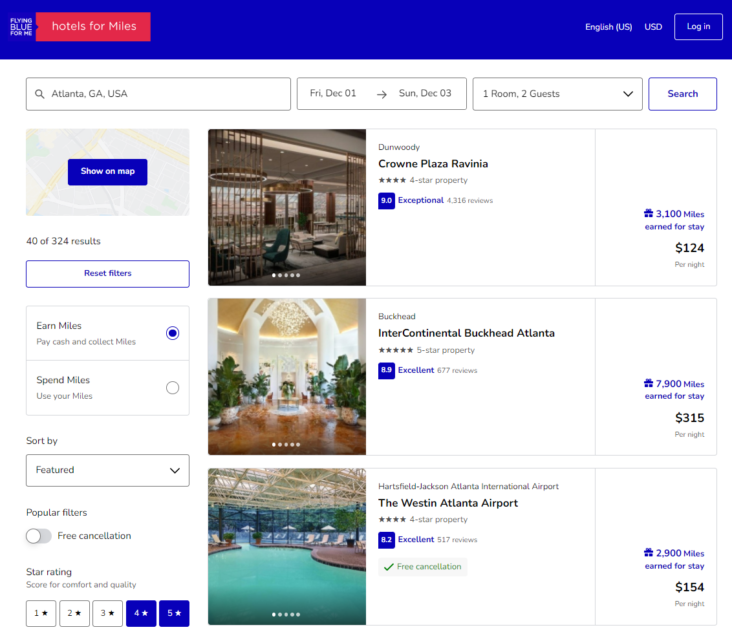The image depicts a smart device or computer screen displaying a hotel search interface. The layout is vertically oriented. 

**Top Section:**
- A blue banner at the top contains the text "Flying Blue for Me."
- To the left, a red box highlights "Hotels for Miles."
- The upper right corner includes options for language (English, US), currency (USD), and a login button enclosed in a small box.

**Search Fields:**
- Below the banner, the background transitions to white, resembling a typical computer screen.
- The search input fields specify:
  1. Location: "Atlanta, Georgia, USA."
  2. Dates: "Friday, December 1st, to Sunday, December 3rd."
  3. Room and guests: "One room, Two guests."
- A prominent search button is available for initiating the query.
- Left of the search button, there is a "Show on Map" link.
- Below these fields, there is an indicator showing "40 of 324 results."

**Filter and Sorting Options:**
- Filters can be reset, and users can choose to earn or spend miles, with "Earn Miles" currently selected.
- Sorting preference is set to "Featured."
- A variety of popular filters are listed, including a toggle for "Free Cancellation" (currently turned off) and star ratings, with four and five-star accommodations selected.

**Results Section:**
- The results are displayed in a list format:
  1. **Dunwoody Crown Plaza Ravina** - Includes rating stars, reviews, and pricing information in both monetary and mile terms.
  2. **Buckhead Intercontinental** - Lists the same details.
  3. **Hartsfield-Jackson Atlanta International Airport, The Westin Atlanta Airport** - Completes the list with similar information.

This detailed layout illustrates how travelers can efficiently search and filter hotels based on various criteria using an online platform.